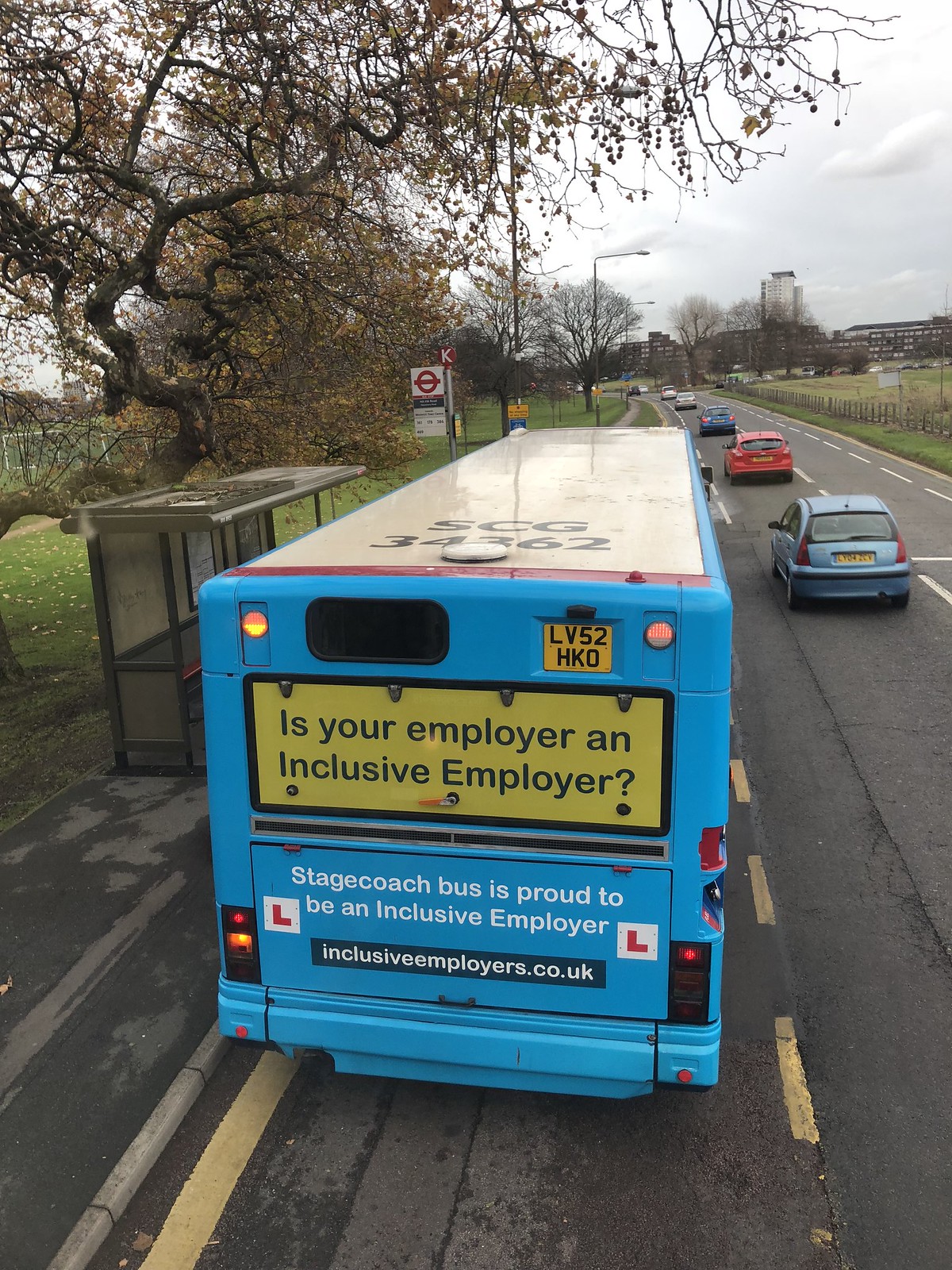The image captures a bird's-eye view of a roadway flanked by a verdant, grassy area on the left with autumnal trees shedding orange leaves, and a bus shelter. On the right, there's a street with cars and another grassy field, extending towards distant buildings under a grey sky. Central to the image is a bright blue bus with a white roof, pulled over in a partial bus lane. The back of the bus features detailed signage: at the top, a license plate with the number LV52HKO, and below, a yellow sign with black text reading "Is your employer an inclusive employer?" Beneath this, a larger black-outlined rectangle contains text stating "Stagecoach Bus is Proud to be an Inclusive Employer," flanked by white logos with red 'L' letters. At the bottom of this rectangle, another box displays the website "inclusiveemployers.co.uk" in white font against a dark background. To the side of the bus in adjacent lanes, there are approximately five cars in various colors: a mid-blue sedan, a red sedan, a deeper blue sedan, and two silver sedans further ahead.